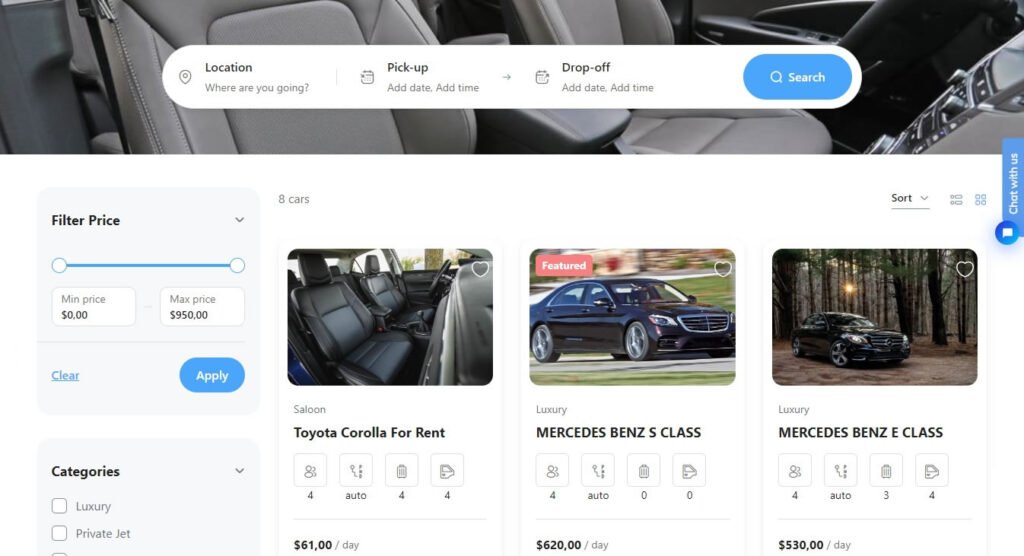This is a detailed and polished caption for the screenshot described:

---

The screenshot displays a sleek car rental website with a minimalist design. The main body of the website features a clean white background. At the top, a wide banner showcases the interior of a car, complementing the site's automotive theme. Centered in this banner is a capsule-shaped white search bar. This search bar consists of four sections: the far left prompts the user to enter a location with the text "Location" followed by "Where are you going?" The next section allows users to specify the pick-up date and time, while the third section is designated for entering the drop-off date and time. On the far right of the search bar, a blue "Search" button stands ready to initiate the query.

Below the banner, the main content area is divided into three columns, each featuring a thumbnail image of a different rental vehicle. On the left side of the page, a pale greyish-blue sidebar provides filtering options. This filter section includes a slider to set the price range, which currently spans from a minimum of $0 to a maximum of $1,950. Options to "Clear" or "Apply" filters are available below the slider. Additionally, there are category options listed, such as "Luxury" and "Private Jet."

The three displayed vehicles are as follows: on the left, a Toyota Corolla is available for rent; the middle column showcases a Mercedes-Benz S-Class; and on the right, a Mercedes-Benz E-Class is featured. Users have the capability to sort the vehicle listings in either a row or grid format, enhancing their browsing experience. There's also a pop-out tab located on the right-hand side of the screen, although its content is not visible in this particular snapshot.

---